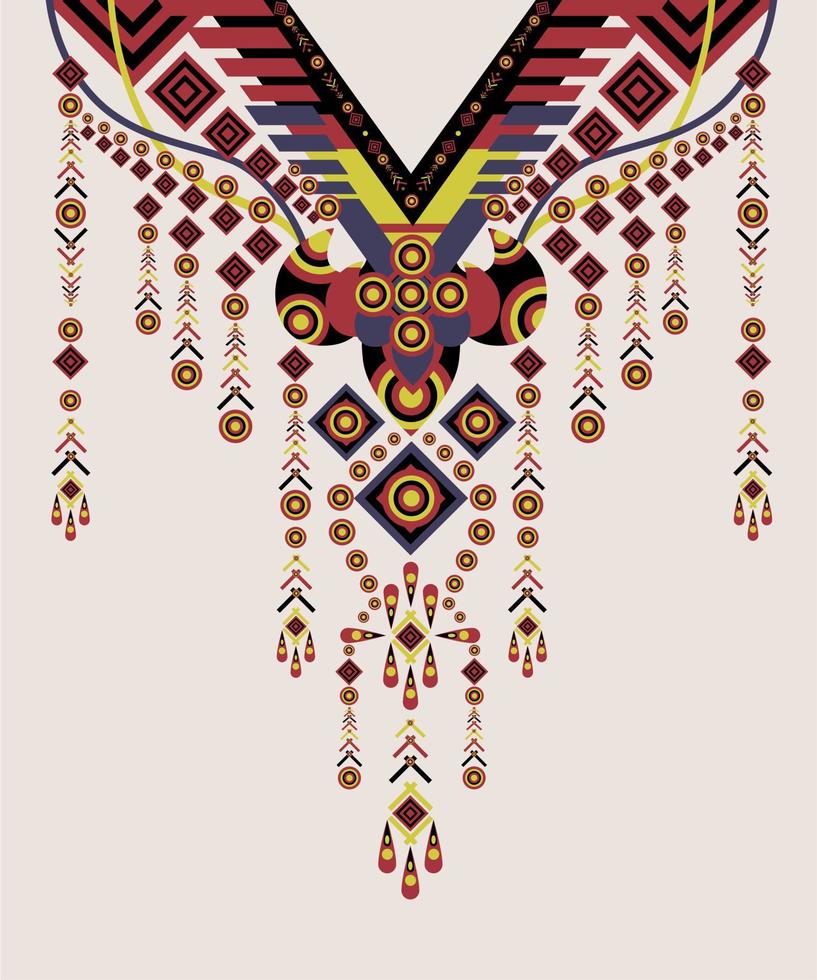The image depicts a highly detailed and colorful drawing on a light background. The design predominantly occupies the upper portion of the image, resembling an elaborate decorative element such as the collar of a Native American style dress or a V-neck on a shirt. At the top center is a black triangular shape, which acts like the apex of the V-neck or collar. This triangular shape is intricately decorated with red and orange circles, diamonds, and small arrows in red and green.

Descending from this peak, the design continues with a series of lines and shapes that hang down, some shorter and others longer, adorned with various geometric patterns. These include red parallelograms, blue parallelograms, and chevrons in multiple colors like yellow, red, and blue. Interspersed among these shapes are a variety of circles, diamonds, and water drop shapes in a diverse palette of colors, including black, yellow, red, and blue.

Towards the bottom of the V, the design features a distinct emblem that resembles the head of a bull. This emblem is composed of a black background filled with concentric circles and dots in red and yellow, further enhancing its intricate and festive appearance. The entire design hangs elegantly, concluding with more chevrons, circles, and diamonds in harmonious repetition, creating a sense of movement and rhythm throughout the piece.

The background of the image is predominantly light gray, with some descriptions suggesting a light pink or off-white hue, adding contrast to the vibrant colors and intricate patterns of the design. Overall, the image is rectangular in shape, taller than it is wide, and measures approximately 5 to 6 inches in height and 4 inches in width. The composition is both decorative and symbolic, evoking a sense of cultural and artistic heritage.